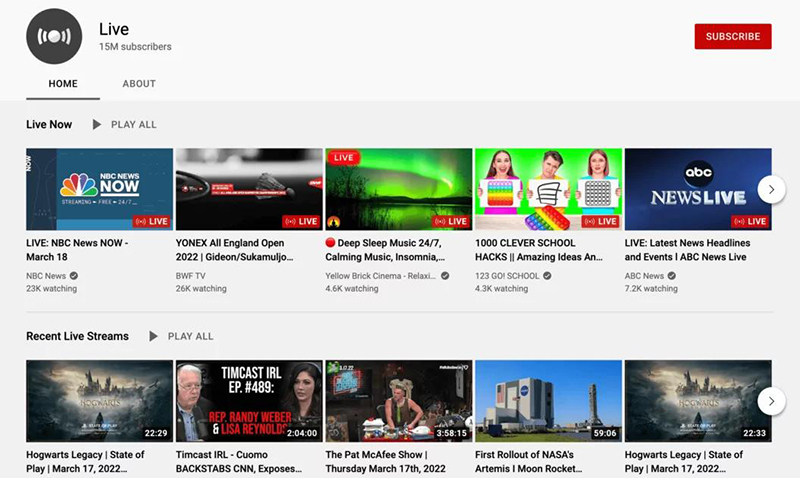In the image, there is a YouTube channel with a grey background featuring several videos. On the top right corner, there's a prominent red "Subscribe" button. The top left displays the channel's icon, which is grey and white. The channel is currently live and boasts an impressive 15 million subscribers. 

Below this, two tabs are visible: "Home" and "About," with "Home" highlighted. Under the "Home" tab, there's a section titled "Live Now," showcasing five live videos:

1. "Live NPC News Now - March 18" by NPC News, with 23k people watching.
2. "Yonex All England Open 2022: Gideon and Soka Mujo" by BWF TV, with 26k viewers.
3. "Deep Sleep Music 24/7 - Calming Music for Insomnia" by Yellow Brick Cinema, with 4.6k viewers.
4. "100 Clever School Hacks - Amazing Ideas" by 123 GO! School, with 4.3k viewers.
5. "Today's Latest News Headlines and Events" by NPC News, with 7.2k viewers.

Further down, in the "Recent Live Streams" section, the following videos are listed:

1. "Hogwarts Legacy State of Play - March 17, 2022"
2. "Timcast IRL: Cuomo Backstabs CNN and Exposes..."
3. "Deep Path - The Cave Shows"
4. "Massive in 2022"
5. "First Rollout of NASA's Artemis Moon Rocket"
6. "Hogwarts Legacy State of Play - March 17, 2022 (repeated listing)"

This detailed organization makes it clear that the channel actively engages its large audience with a diverse array of live content.